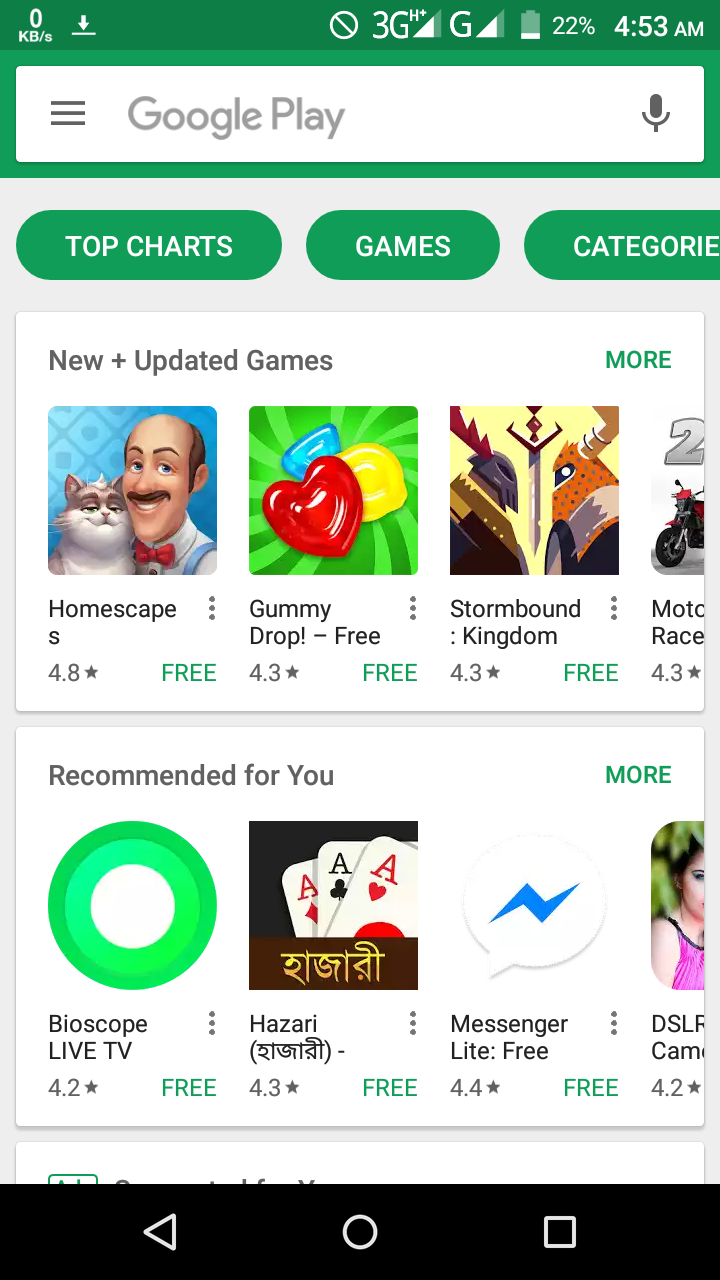Screenshot of a mobile device displaying the Google Play Store interface. The screen shows the Google Play Store app with a dark green navigation bar at the top, featuring white text that reads "Google Play." The bar contains a menu icon on the left and a microphone icon on the right. The status indicators reveal that the device is connected to a 3G network, has a battery level of 22%, and the current time is 4:53 AM. 

Below the navigation bar is a pale gray or white background with three green headers labeled "Top Charts," "Games," and "Categories." These headers are in the form of oblong green ovals. Underneath, there's a white text box titled "New and Updated Games," with a "More" link to the right.

The games section features square thumbnail images for different games:
1. **Homescapes**: Depicts a mustachioed bald man holding a smiling cat, rated 4.8 stars, and listed as free.
2. **Gummy Drop!**: Shows colorful gummy candies, also free.
3. **Stormbound: Kingdom Wars**: Features cartoon-style Viking or medieval armored characters, partially cropped.
4. Another game with a thumbnail that is cut off, showing part of a motor or mechanical element.

Further down, another white text box labeled "Recommended for You" appears with a "More" link on the right. The recommended apps include:
1. **Bioscope LIVE TV**: Rated 4.2 stars, and free.
2. **Hazari**: Contains Sanskrit or Hindi text, rated 4.3 stars.
3. **Messenger Lite**: Rated 4.4 stars, and free.
4. An app related to DSLR cameras, cropped off and partially visible.

The overall screenshot encapsulates a typical browsing experience on the Google Play Store during the early hours of the morning.